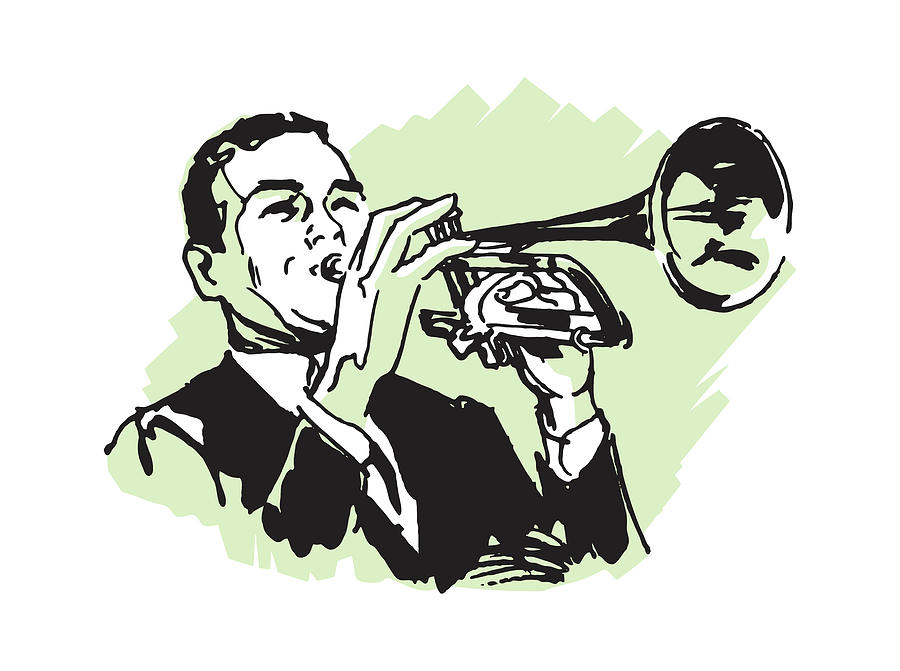A simple and visually striking illustration features a man deeply immersed in playing a trumpet. The cartoon-style drawing primarily uses three colors: black, light green, and white. The man is dressed in a black suit jacket over a white button-down shirt with a tie, exuding a formal yet passionate demeanor. His face is highlighted in white, with the rest of his skin in a light mint green shade. The background, also adorned with light mint green brush strokes, complements his appearance. The man's hands are skillfully positioned on the trumpet—right hand manipulating the three keys on top, left hand supporting the instrument from the bottom. His absorbed expression suggests he's playing from memory, underscoring his musical talent and expertise. This clean and focused illustration captures both the elegance and intensity of the musical moment.